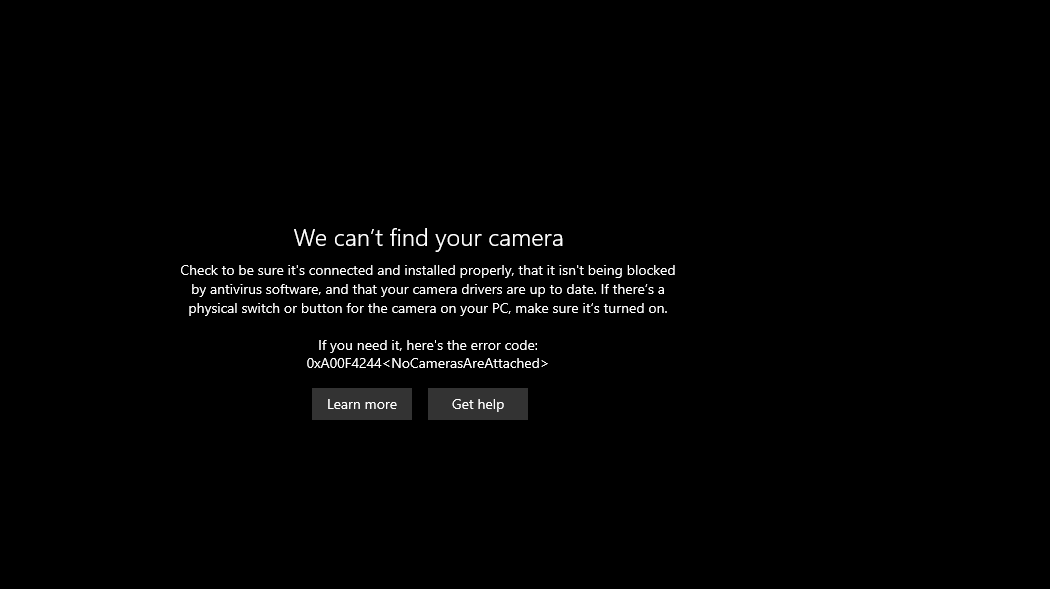The image features an entirely black rectangle serving as the background. Centrally aligned but slightly left of center, the primary text appears in a bold, larger font stating: "We can't find your camera." 

Below this, in smaller font, the instructions read: "Check to be sure it's connected and installed properly, that it isn't being blocked by anti-virus software, and that your camera drivers are up to date. If there's a physical switch or button for the camera on your PC, make sure it's turned on."

Following a line break, the message continues, "If you need it, here's the error code:" 

Directly below, the error code "0xA00F4244<NoCamerasAreAttached>" is displayed prominently. 

At the bottom of the image, two buttons labeled "Learn more" and "Get help" appear in white text.